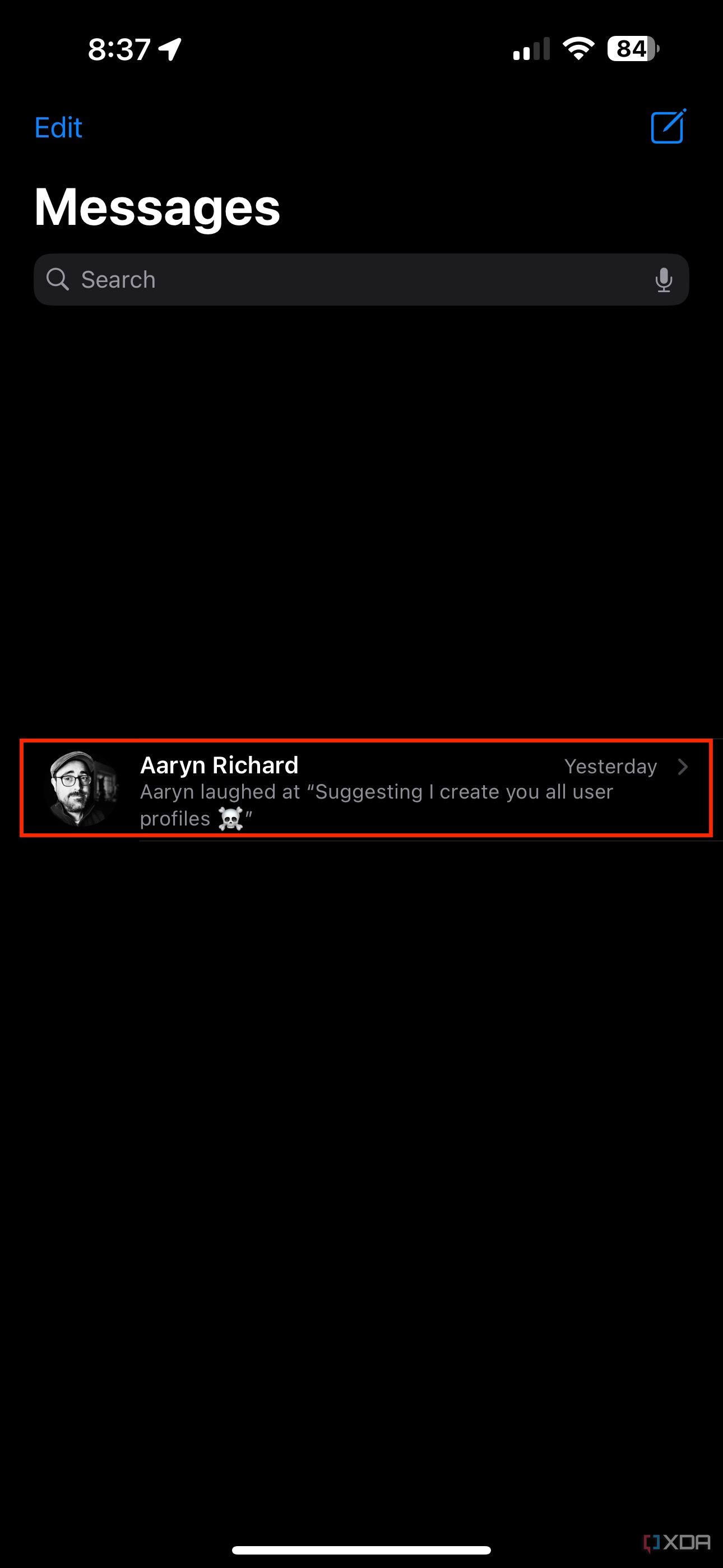A detailed screenshot of an iPhone Messages app is captured. At the top of the screen, large white letters proclaim "Messages." Below this header is a search bar extending from the left to the right edge of the screen, containing the word "Search," flanked by a magnifying glass icon on the left and a microphone icon on the right.

Centered within the message list, one message is visible amidst blacked-out sections. The sender's profile picture appears on the left. To the upper right of the profile picture is the sender's name, with the actual message displayed directly underneath. In the top right corner of this message entry, "Yesterday" is noted, accompanied by a right-pointing arrow icon. 

A red box has been added to the image, emphasizing this particular message. In the bottom right corner of the screenshot, a small "XDA" logo is visible.

Further details present at the top of the screen include: on the left, "Edit" in small blue lettering, and on the right, an icon depicting a piece of paper with a pen, indicating the option to start a new message. The status bar at the very top includes the time on the left, along with a location icon. The right side of the status bar displays a phone signal icon, a Wi-Fi icon, and a battery percentage icon.